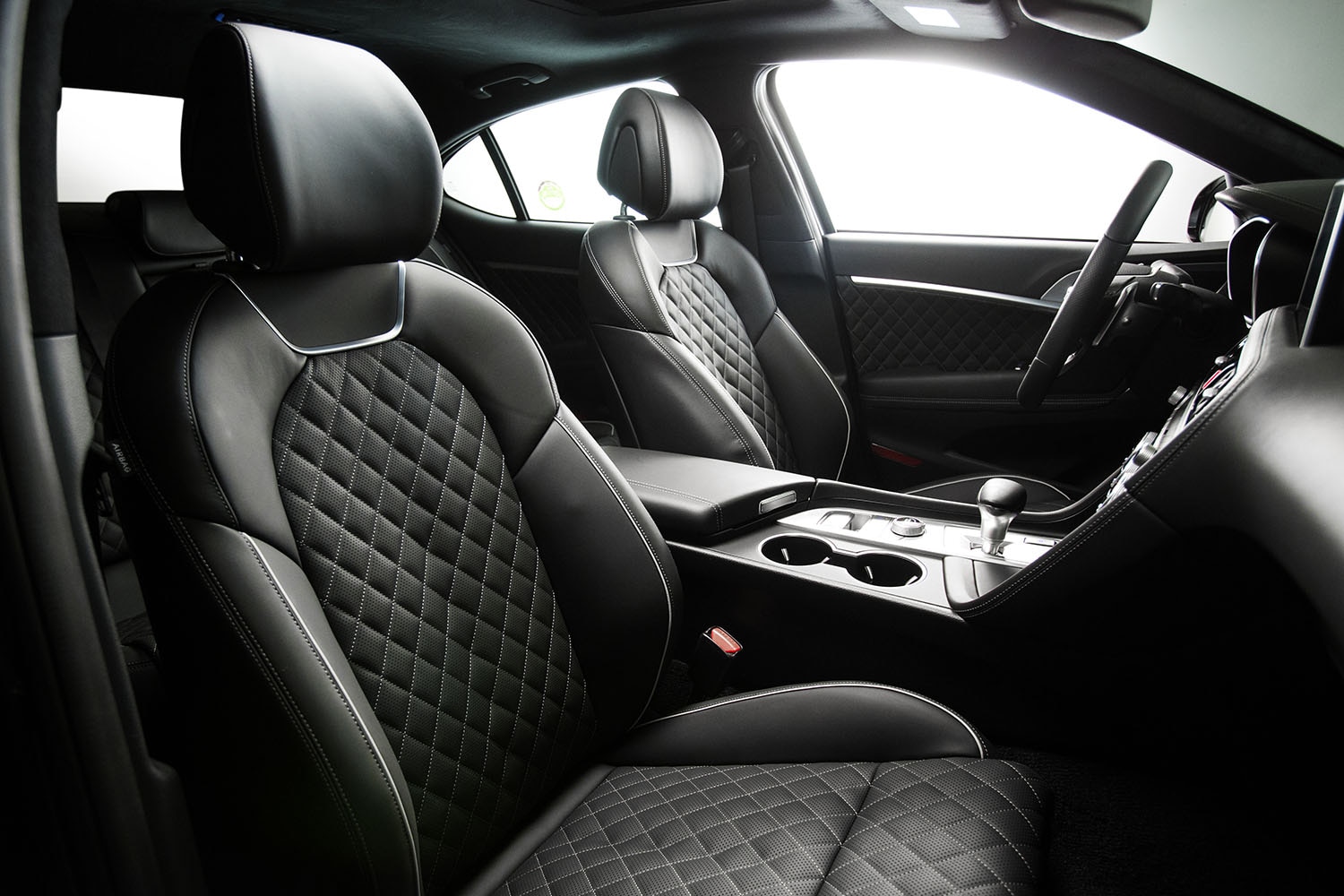This image captures the interior of a modern luxury car from the perspective of the passenger seat looking towards the driver's seat, both of which are empty. The car boasts an entirely black leather interior accentuated by distinctive white stitching that forms a checkerboard or diamond pattern, notably down the middle of each seat. 

The front seats, along with the equally pristine back seats, show no sign of wear, underscoring the car’s brand-new condition. The center console, finished in silver, houses two cup holders and a multifunctional storage compartment. 

A large, prominent steering wheel dominates the driver’s area, suggesting ease of control. The vehicle's automatic gear shift enhances its modern appeal. Though primarily black, the interior features subtle red accents, including a small compartment at the bottom half of the door. 

The vehicle is a four-wheel drive, illuminated by a bright, white light from outside which pours through the three driver’s side windows, rear window, and the front windshield, providing high visibility within the cabin.